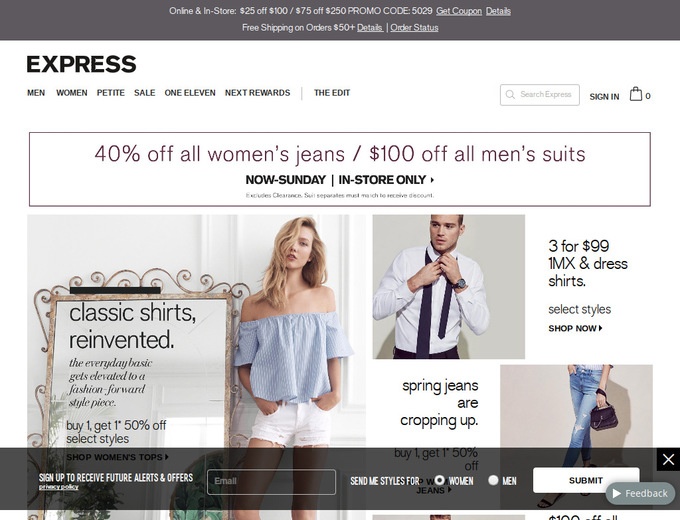This is a screenshot of the Express shopping site. At the very top, a wide grey bar displays various promotional offers including "$25-$100 off," "$75 off $250," among other details. Below this bar, the main navigation menu offers categories such as "Men," "Women," "Petite," and "Sale," with a search bar located on the right side. 

A prominent banner stretches across the page announcing "40% off all women's jeans and 100% off all men's suits," valid in-store only from now through Sunday. The center of the image features a woman wearing a light blue top and white shorts. To her right, a man is shown tying a tie around his white shirt, and another woman on the far right is wearing a pair of jeans. On the far left, there is a standing gold-framed mirror, reflecting the text "Classic Shirts Reinvented."